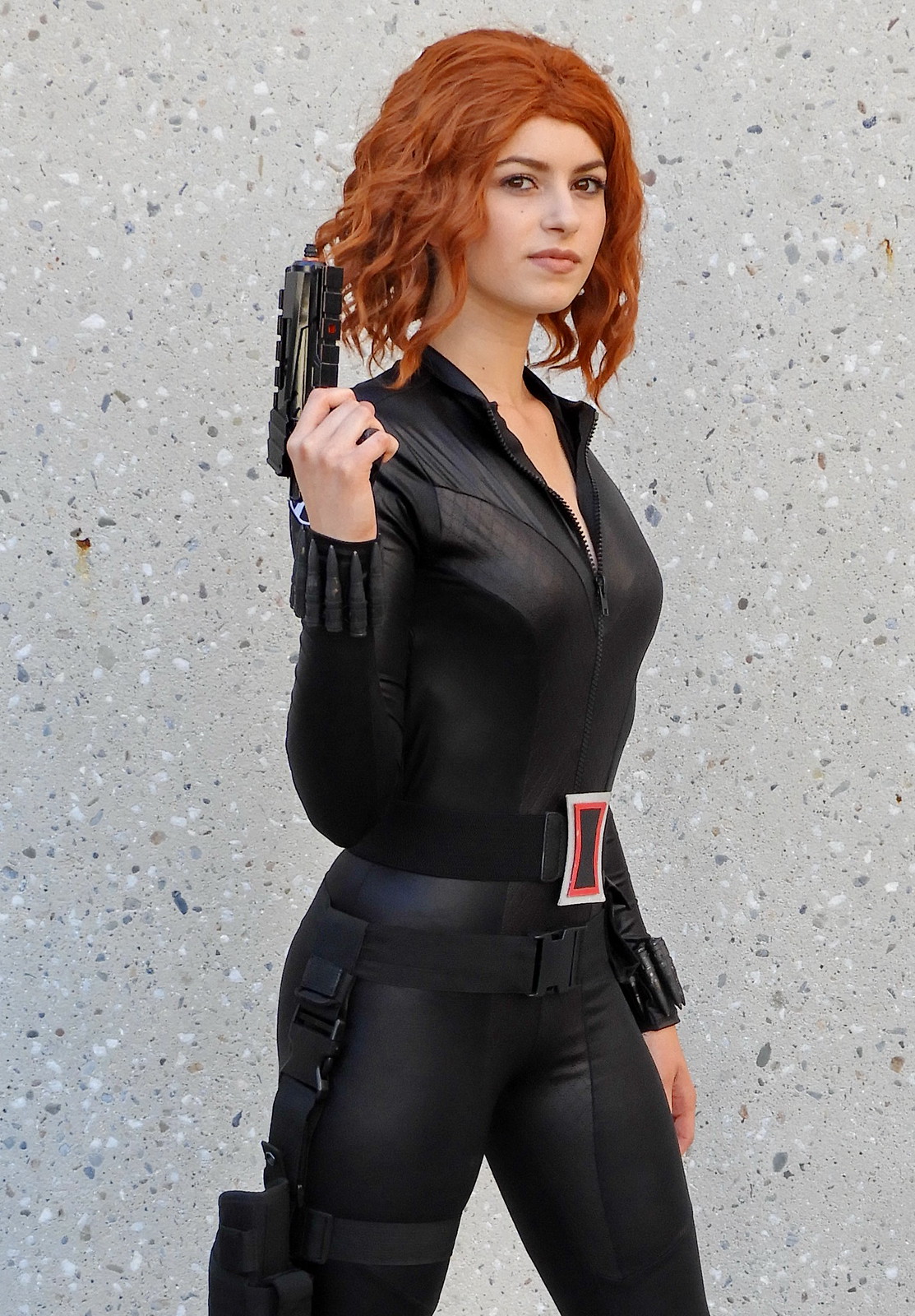The photograph captures a young woman in an elaborate cosplay outfit, possibly portraying a character from Disney or Marvel. She wears a conspicuous red auburn curly wig styled in a poofy bob that looks slightly awkward. Her attire is a skintight, long-sleeve black leather bodysuit with a front zipper, accentuated by belts and straps. A belt around her waist features a distinctive red, black, and white square buckle, and additional belts and holsters adorn her right leg. Her right hand grips a black gun, while bullets are affixed to the cuffs of her sleeves on both arms. She stands confidently in front of a gray and white speckled wall, with her left leg positioned forward and her right leg extended back. Her right arm is raised with the gun, and her left arm rests at her side. She gazes directly at the camera, embodying the character she portrays with a deliberate and engaging stance.